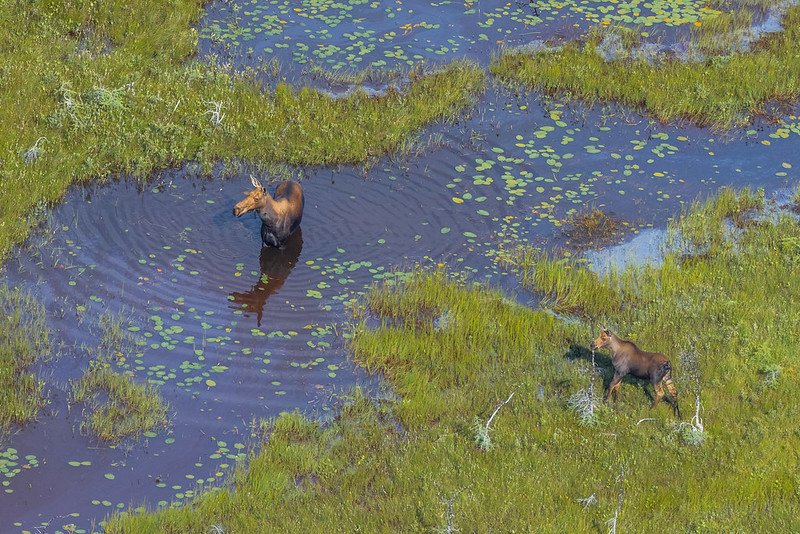Two moose are captured in this overhead aerial photograph, set within a vibrant marshland. Taken by a drone, the image provides a detailed view of the wet, grassy environment. The central section of the photo is occupied by clear, dark blue water, dotted generously with green lily pads. One of the moose, a dark brown adult, stands partially submerged in this water, its dark coat appearing nearly black from being wet. It seems to be drinking while also alertly looking to the left, perhaps reacting to the drone or something else just out of frame. Towards the bottom right, walking through the bright green, swampy grass interspersed with white tree limbs, is a smaller moose. This moose is dark brown underneath with a lighter brown top and light tan inner back legs, also turning its head to the left. The scene captures the serene yet vigilant mood of the two moose in their natural habitat.